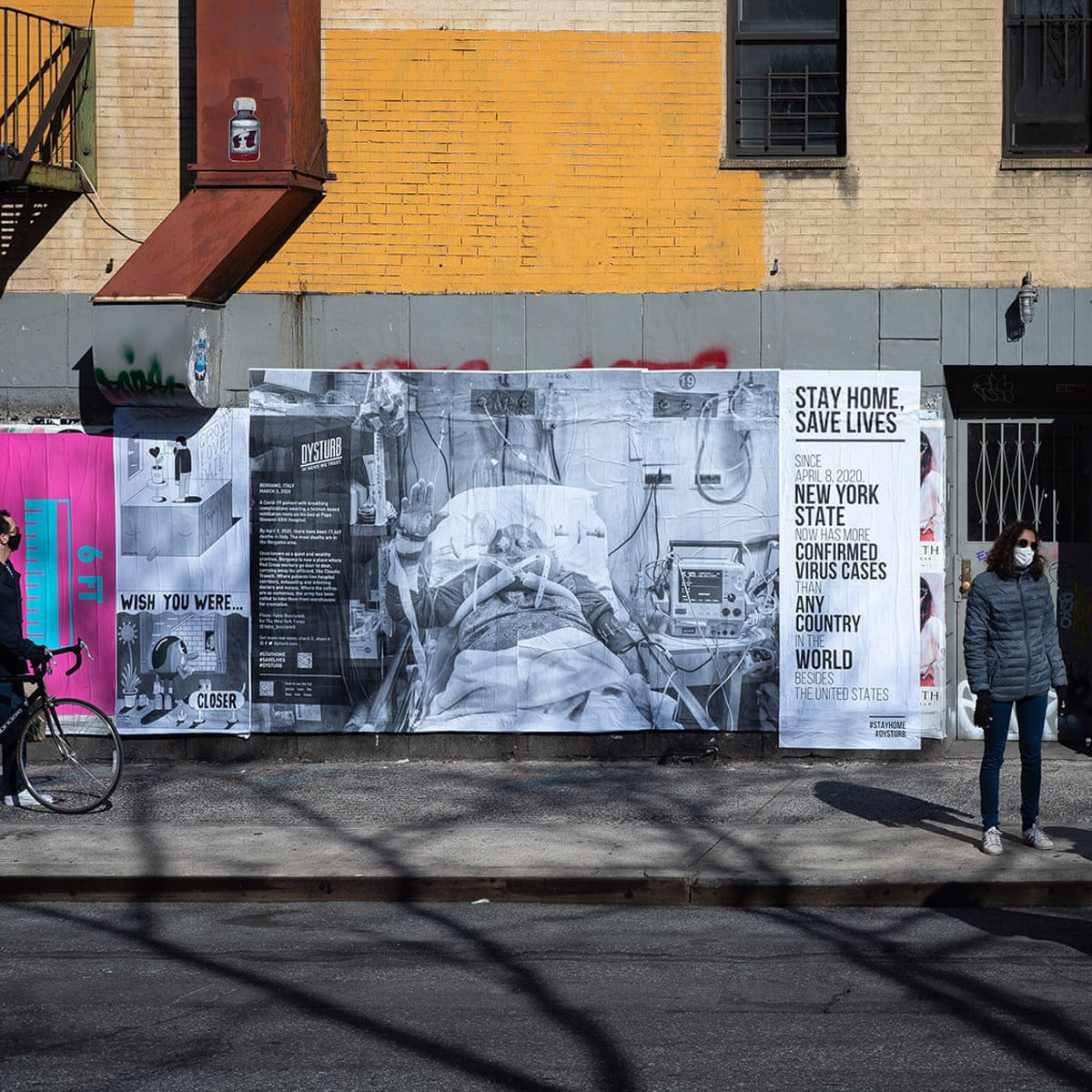The photograph captures a bustling city street scene, dominated by an imposing black and white notice affixed to the side of a building. At the center of the notice, a striking image shows a person lying in a hospital bed, connected to an array of medical machines, with their right arm raised. Above this poignant visual, bold black text commands, "Stay Home, Save Lives." Below the image, a grim statistic reads, "Since April 8, 2020, New York State now has more confirmed virus cases than any other country in the world besides the United States." Another piece of related text on the notice poignantly states, "Wish you were closer."

The backdrop reveals a brick building, partially painted yellow, with barred windows. The street scene includes a woman on the sidewalk, who is dressed in black pants, a gray coat, white face mask, and sunglasses. With her black bob haircut and facing the camera, she embodies the caution of the times. To the left, partially visible, is a man walking his bike, glancing up at the towering billboard, evoking a sense of solemn recognition. Both individuals are navigating the constrained urban space, their presence adding a human touch to the stark and somber public health message.